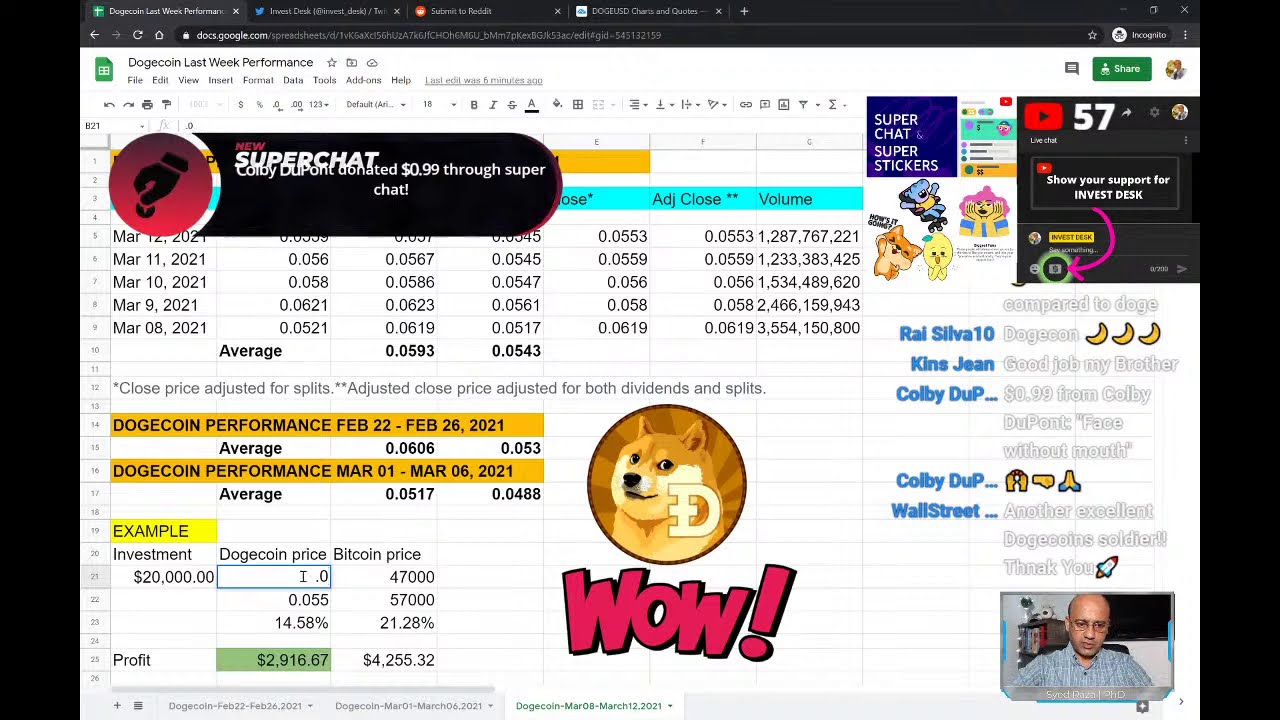The image displays a computer screen showing a webpage designed to track Dogecoin performance, resembling a spreadsheet or financial chart. The page features a black banner near the top labeled "Super Chat" with a red circular logo. Below, several columns of data indicate "Volume," "A," "D," "J," and "Close," likely representing Dogecoin metrics for February and March. Central to the page, an animated dog within a black-outlined circle, with a white "D" over the image and "WOW!" in bold red text beneath it, signifies Dogecoin. The layout also includes performance graphs and a list of prices, dates, and volumes, suggesting a stock or commodity tracking setup akin to Wall Street displays. On the right-hand side, symbols and names appear, along with a small frame of a man seemingly involved in an online chat, facing the viewer with a monitor visible over his left shoulder. The webpage is bordered on the left and right by black bars, housing additional symbols and text related to the site's address and functions.